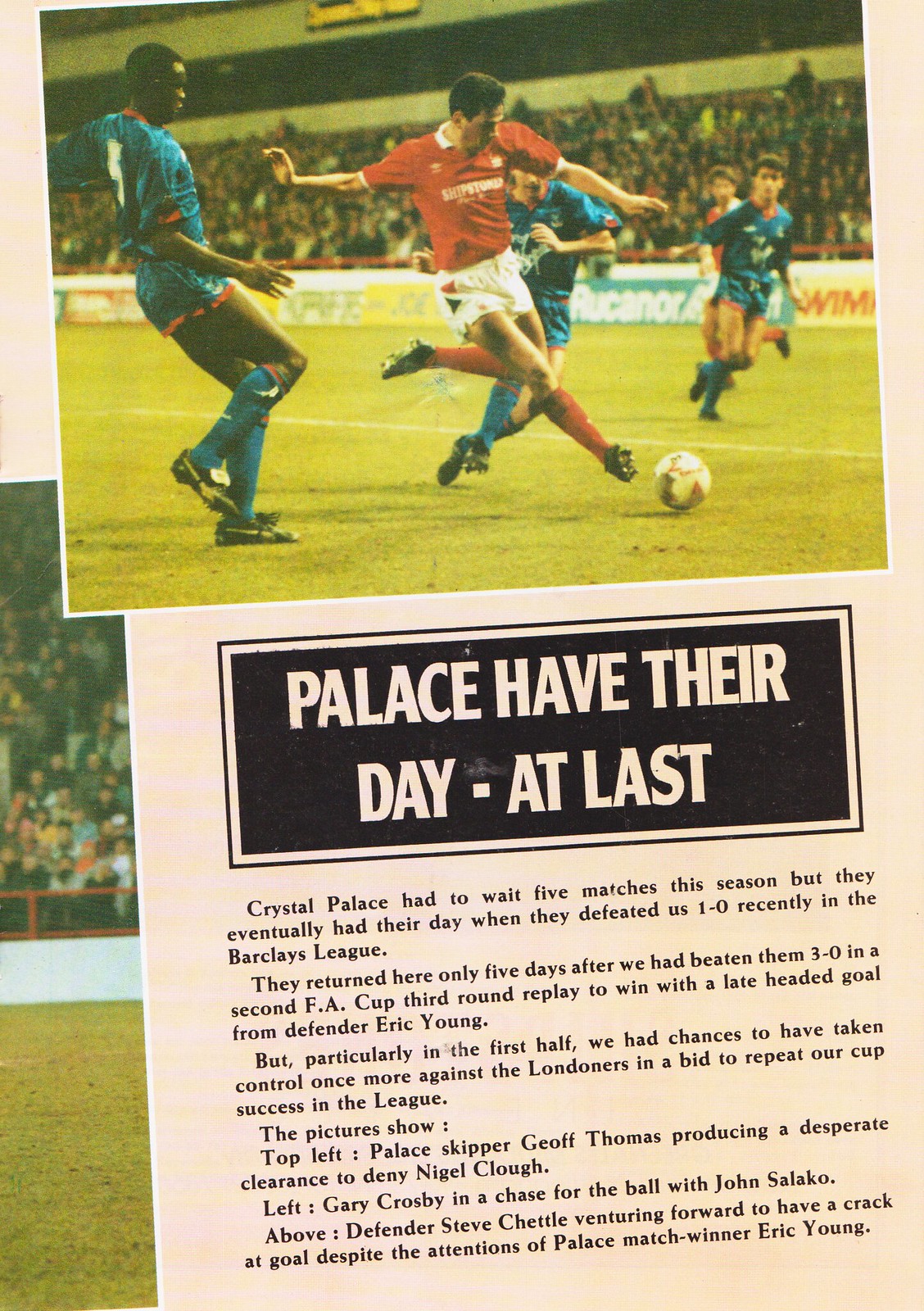The image features a slightly tilted, rectangular photograph at the top, displaying an intense soccer game. The scene captures five players: three in blue jerseys and two in red. A player in red is about to kick the ball while surrounded by blue team members, set against a green turf field with a packed stadium in the background. Beneath this action shot, a pink-colored poster titled "Palace have their day at last" is prominently displayed, also tilted slightly to the left. The poster details Crystal Palace's recent 1-0 victory over their rivals in the Barclays League, a triumph achieved with a late headed goal by defender Eric Young. The text narrates how Palace overcame previous defeats, including a recent 3-0 loss in the FA Cup replay. Descriptions within the article highlight key moments, such as Palace skipper Jeff Thomas's critical clearance to deny Nigel Clough and defender Steve Chettle's offensive attempts despite Eric Young's defense. On the left side of the image, another photograph is partially visible, showing a segment of a sports field and spectators in the stands. The remaining background of the image is predominantly pink, adding to the vibrant and dynamic feel of the composition.